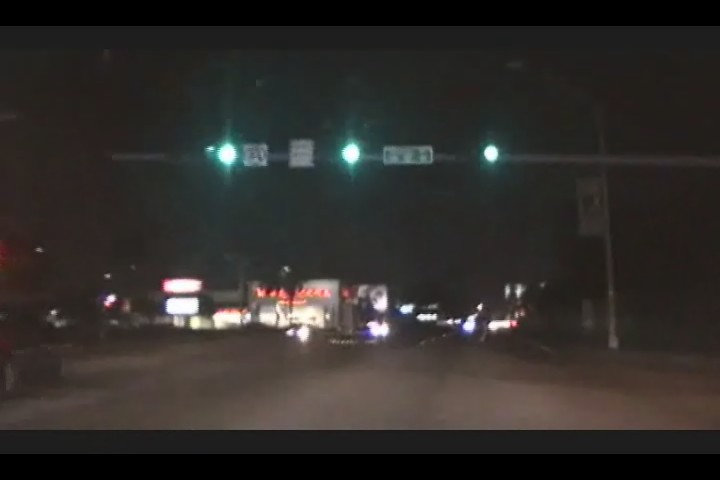A blurry nighttime photograph likely taken from a moving vehicle's perspective shows an intersection illuminated by three green traffic lights supported by a vertical post. The edges of the image are dark black, fading into a gray border underneath. To the left, there is a black SUV, blurred as if in motion. A light pole on the corner has its light out, contributing to the dim ambiance.

The intersection is marked by white lines ahead but none in the center. The road surface is gray concrete. In the background to the left, a store with red neon signs is partially obscured by a tree. Other buildings and oncoming car lights add to the bustling yet indistinct urban night scene. The overall blur and slight tilt suggest the photo was captured from a moving vehicle, possibly a dash or night cam, emphasizing the sense of motion and dynamism in a nighttime cityscape.